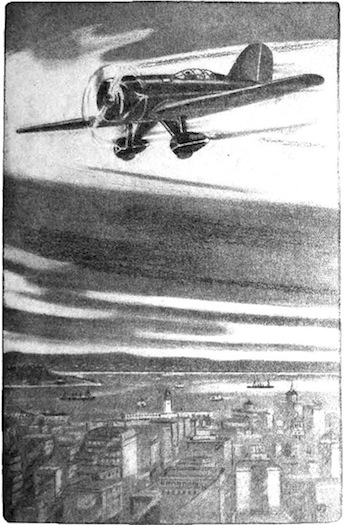The image is a black-and-white drawing titled "Viking of the Sky" by Hugh McAllister, depicting an old, single-pilot airplane soaring high above a sprawling cityscape. The airplane, reminiscent of those used for crop dusting with its long wings and front propeller, is positioned at the top of the image, surrounded by billowing clouds that contribute to a dynamic sense of motion. Below, an expansive city is detailed with various buildings seen from above, including a lighthouse. Beyond the city, a body of water stretches out, populated with at least five boats of varying sizes, some appearing as sailboats. The scene's backdrop features rolling hills or mountains, adding depth to the composition. The drawing captures the bustling energy of the city and the tranquil expanse of the water and hills, all beneath a cloud-streaked sky.